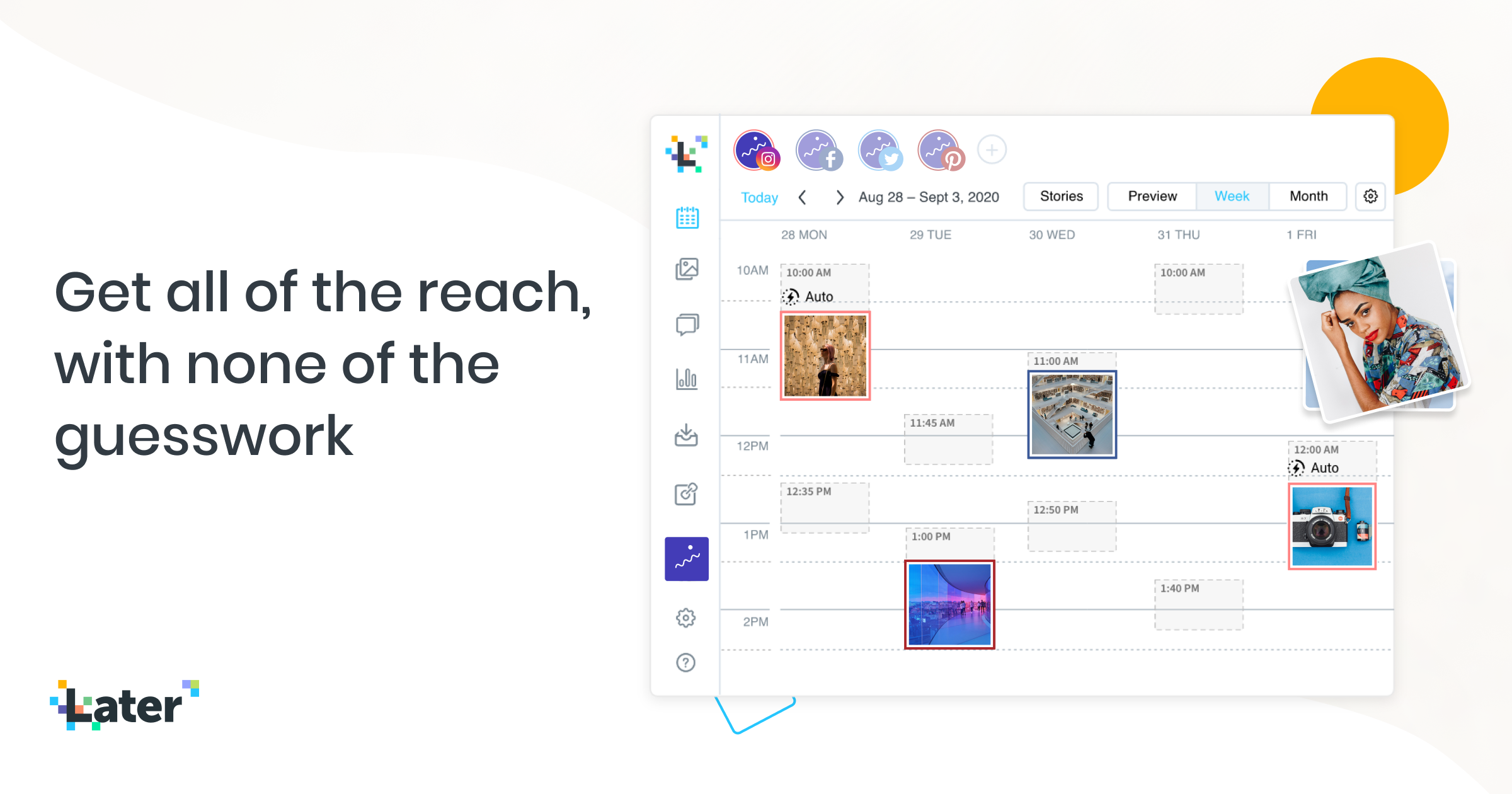This is a detailed screenshot of a promotional webpage for the website "Later." On the left side of the screenshot, there is bold black text that reads "Get all the reach with none of the guesswork." At the bottom left corner, the word "Later" is displayed, indicating the name of the platform being advertised.

The right side of the image shows a mockup of the website's interface. At the top left, the Later logo is prominently featured, depicted as a stylized "L" surrounded by pixelated dots in various colors, including yellow, green, and blue. This area emphasizes the branding of the platform.

Directly below the logo, there are icons for several social media platforms, including Instagram, Facebook, Twitter, and Pinterest, suggesting that Later specializes in social media integration and management.

Further down, there is a section labeled "Today" as well as a date range reading "August 28th through September 3rd, 2020." Beneath this, a calendar layout is visible, detailing different events scheduled between 10 a.m. and 2 p.m., illustrating Later’s functionality in planning and organizing social media posts and activities.